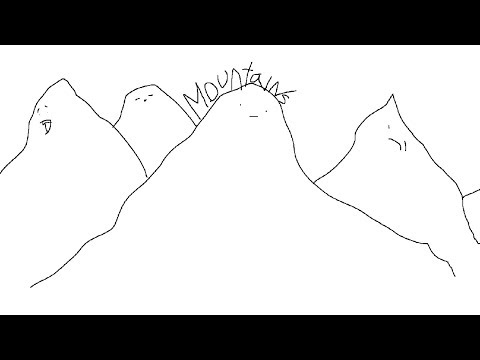This is a hand-drawn, black pen or marker illustration on a white background, depicting four simplistic, cartoonish mountains. Each mountain is cone-shaped with a face at its peak. The first mountain on the left has an open mouth, giving it an expressive look. The second mountain from the left, which appears in the background, features a basic face with two eyes and a small dot for a nose, resembling closed eyes or a sleeping expression. The third mountain stands prominently in the foreground with handwritten, slightly sloppy text that reads "mountains" written above it; its face displays two dots for eyes and a straight line for a mouth, suggesting a neutral or confused demeanor. The fourth and final mountain on the right has a slanted face that looks distorted or sad. Additionally, the drawing is bordered by black bars at the top and bottom, framing the simplistic yet whimsical depiction.